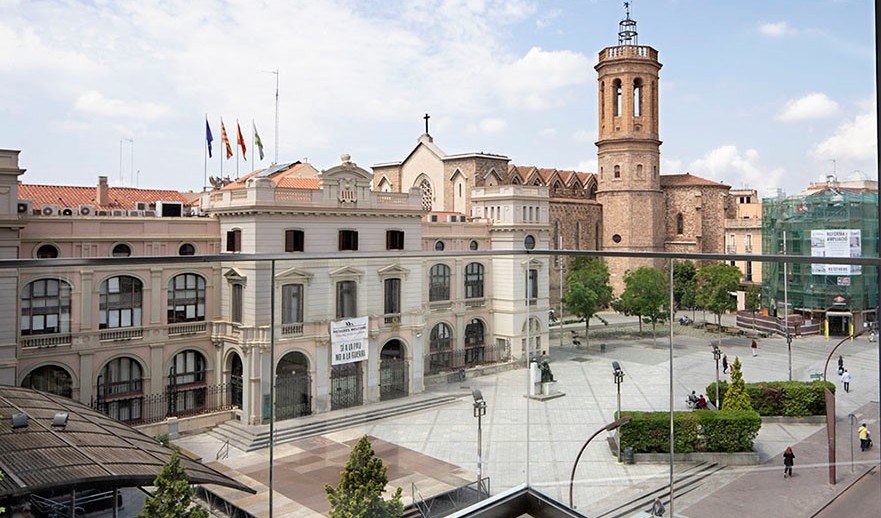The image depicts a clean and crisp courtyard set in a European city, likely in France, characterized by a blend of historical and modern architecture. The courtyard is surrounded by a range of buildings: beige and white with some brick, evoking a sense of longstanding European architecture. In the foreground, to the left side, there are tall hedges and lampposts aligning with steps and a few people scattered, enjoying the scene but not crowding the area. The cloudy sky adds a soft light to the scene, indicating it might be spring or summer. 

Prominent in the courtyard is a black statue, with seating arrangements nearby. A collection of colorful flags and banners, though unreadable, add vibrancy to the scene. The left side of the courtyard hosts older, tan-colored buildings, while the back-right features a newer, green glass building, creating a striking contrast. A church or possibly a cathedral with brownish-tannish brickwork is also visible, hinting at the historical depth of the area. The image suggests an official or business district, with serene activity levels and an aesthetic mix of tradition and modernity.